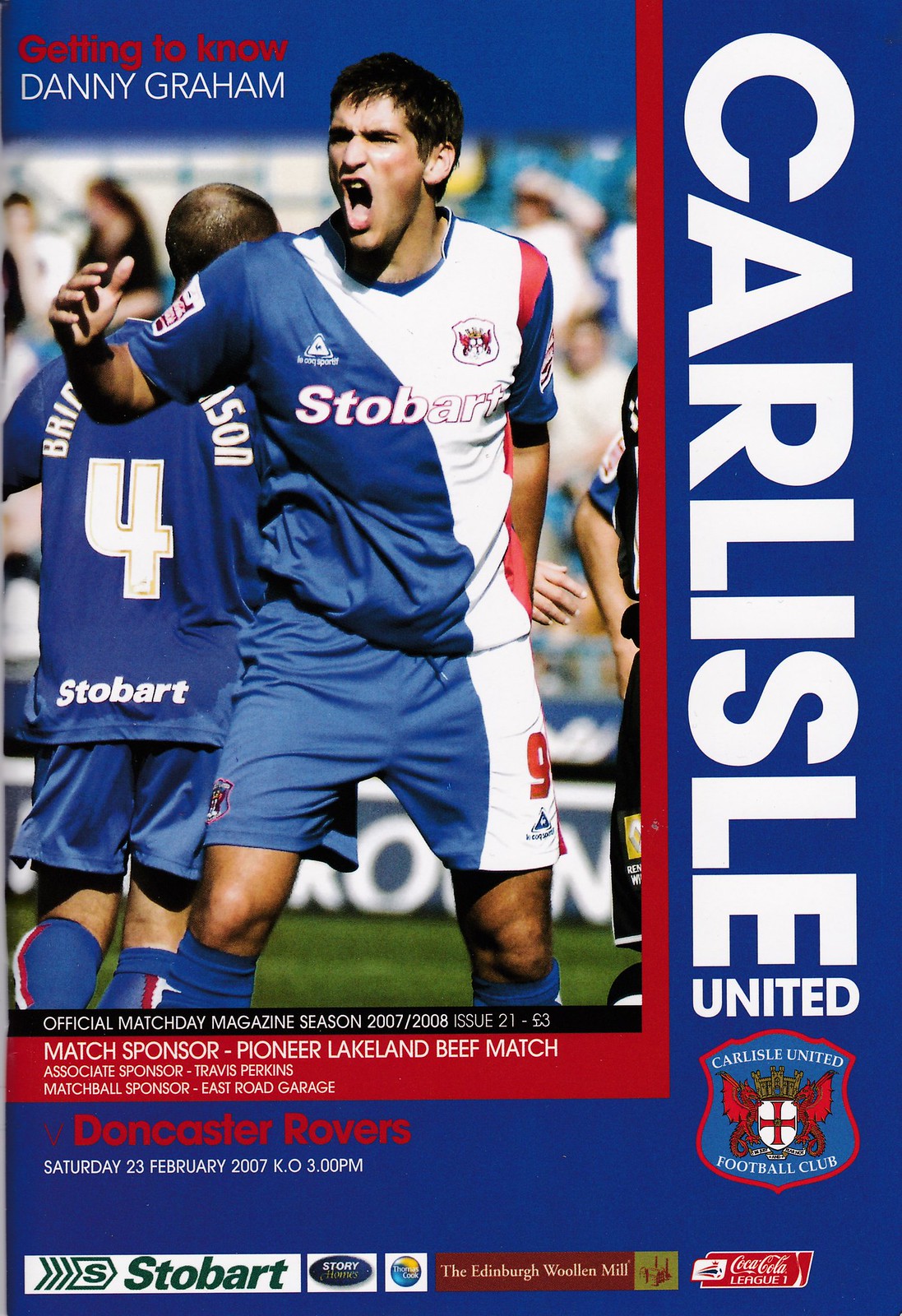The image is a full-color cover of an official soccer program, likely a portrait or magazine cover featuring an athlete named Danny Graham. The large photograph of the soccer player dominates the upper left portion of the cover, showing him with an intense expression, mouth open as if yelling. Danny Graham, identified by the text "Getting to Know Danny Graham" prominently displayed on the cover, is dressed in a soccer uniform in blue with white and red stripes, indicating his association with Carlisle United, as denoted by the text stretching vertically on the right-hand side. The program is for a match between Carlisle United and Doncaster Rovers, set for Saturday, 23 February 2007, at 3:00 PM, as indicated on the cover.

Additional text under Graham's picture details its broader context: "Official Match Day Magazine, Season 2007-2008, Issue 21-53, Match Sponsor Pioneer Lakeland Beef Match, Associate Sponsor Travis Perkins, Match Ball Sponsor East Road Garage." There is also a logo for Carlisle United Football Club located at the bottom right corner. The overall design includes a color palette of peach, black, brown, red, white, and blue, enriching the professional and athletic feel of the cover.